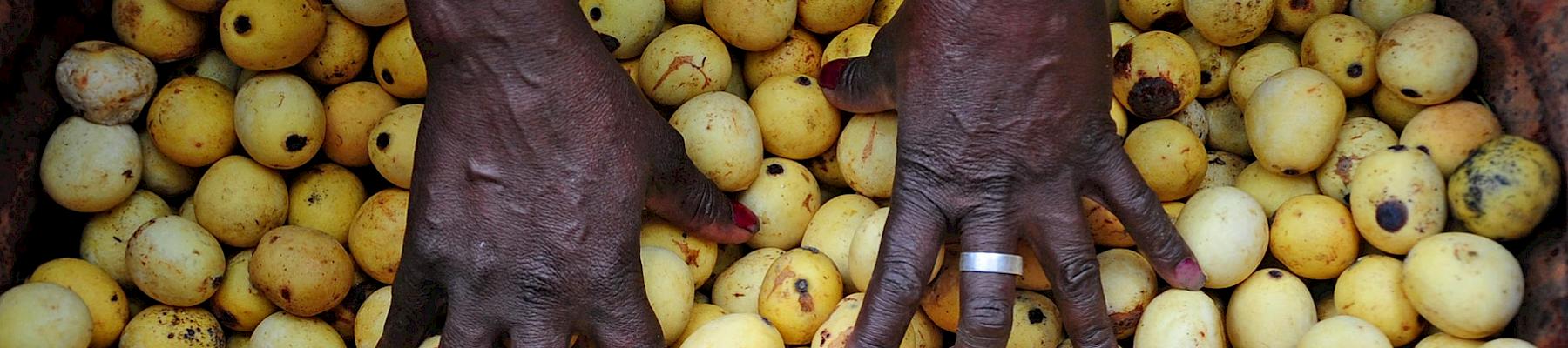This photograph features a pair of African-American hands, seen from above, delicately placing or assessing a collection of oval, egg-shaped objects in a container. The hands, dark chocolate in color, display prominent veins and belong to an individual wearing a distinctive silver ring on the middle finger of the left hand. The container holds a variety of items that appear to be either potatoes or a type of yellow fruit, with some exhibiting a white, yellowish-brown hue and others showing brown splotches, possibly indicating spoilage. The composition of the image is horizontal and thin, focusing intently on the hands and the mysterious produce they touch, highlighting the texture and color contrast between the hands and the items in the container.